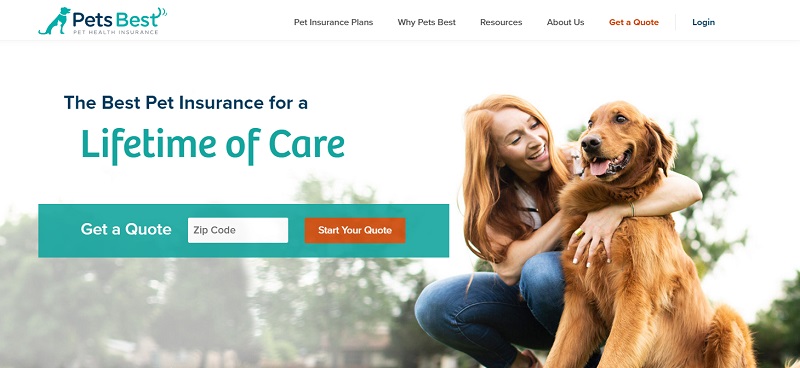The image appears to be from a website with a white background. In the top left corner, there is a logo featuring a picture of a dog accompanied by the text "Pet's Best Pet Health Insurance." Moving to the right, there are several navigation options: "Pet Insurance Plans," "Why Pet's Best," "Resources," "About Us," and "Get a Quote." A thin gray line separates these options from a "Login" button.

Below this, on the right side of the advertisement, there is a charming picture of a happy brown dog with its tongue playfully sticking out. Beside the dog, a woman is crouching down, smiling broadly, and hugging the dog warmly. To the left of this heartwarming image, text reads, "The Best Pet Insurance for a Lifetime of Care," followed by a call-to-action button labeled "Get a Quote." Beneath this button, there is a field for entering a zip code, accompanied by another button that says "Start Your Quote."

In the background of the overall image are lush green trees, adding a touch of nature and tranquility to the scene.